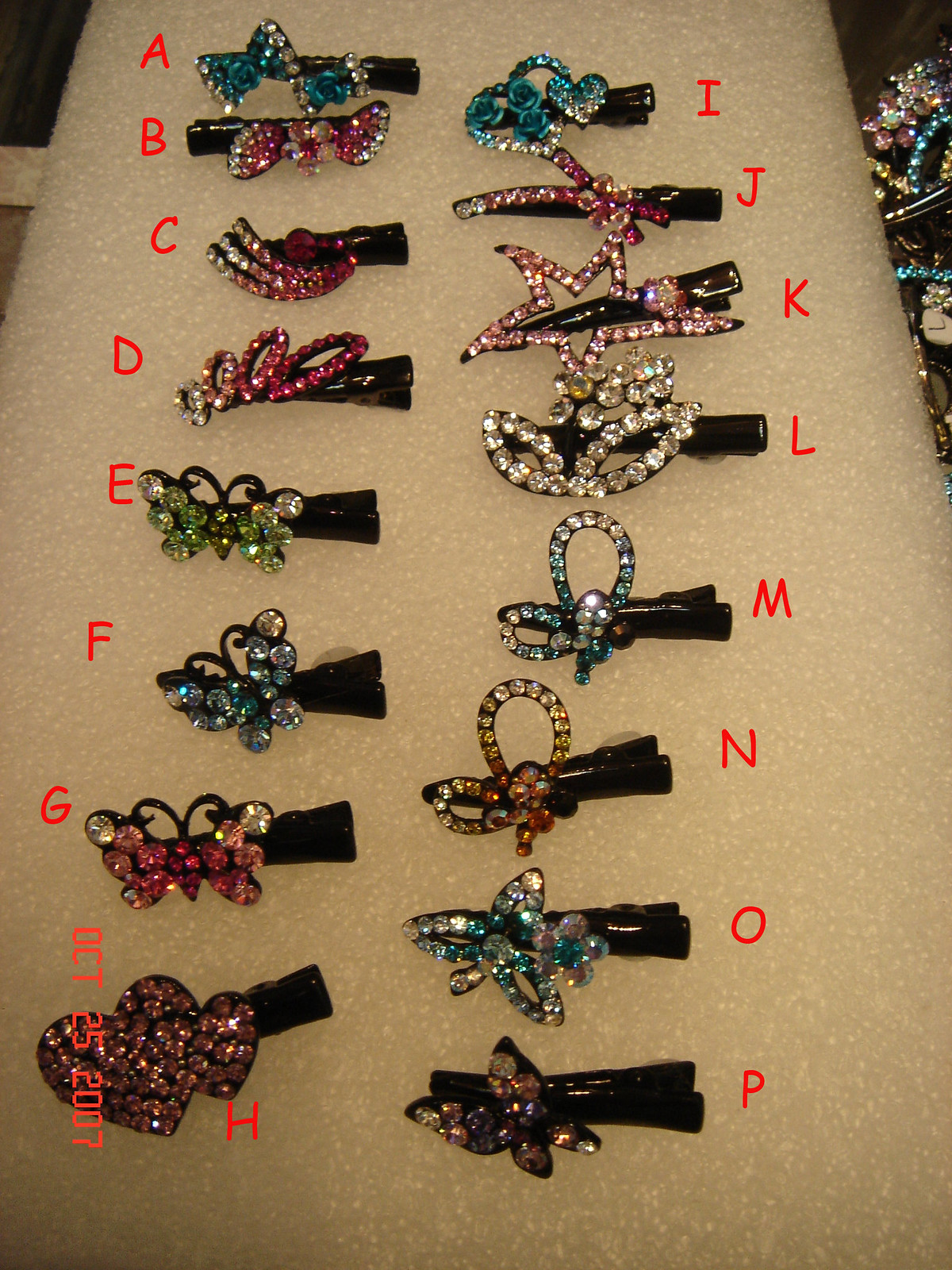This is a vertical, color photograph dated October 25, 2005, displaying a collection of intricately designed rhinestone hair clips arranged neatly on a styrofoam board. The hair clips are labeled with red letters from A to P, and they are positioned horizontally with the clip parts pointing toward the right. Each clip, set on a black post, features dazzling rhinestone designs in various shapes and colors including blue and white bows, pink crowns, green and blue butterflies, purple hearts, gold bows, pink stars, and blue hearts adorned with little roses. The clips are displayed in two vertical rows against a cream-colored, foam-like background, highlighting their elegant appearance and intricate detailing.